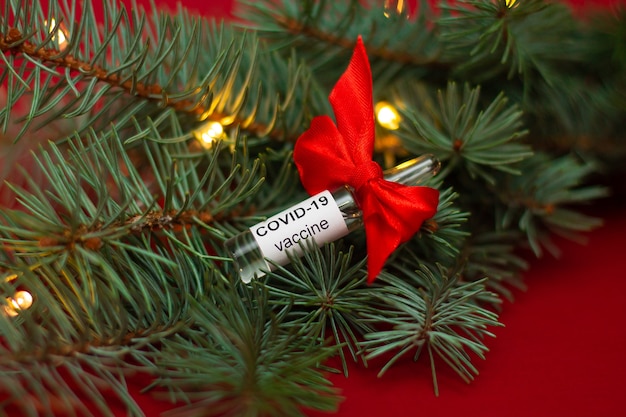The photograph captures a festive scene featuring a small glass vial labeled 'COVID-19 vaccine' in black sans serif font on a white background. The vial, lying diagonally across the photo, has a tiny red Christmas bow tied around its upper part, just below the cap. Surrounding the vial are green branches typical of an evergreen Christmas tree, adorned with glowing yellow Christmas lights. The branches and the vaccine vial rest on a red surface, possibly fabric, adding to the holiday-themed setting. This creates an imagery symbolizing the COVID-19 vaccine as a precious gift to the world, aligning with its release around the Christmas season.